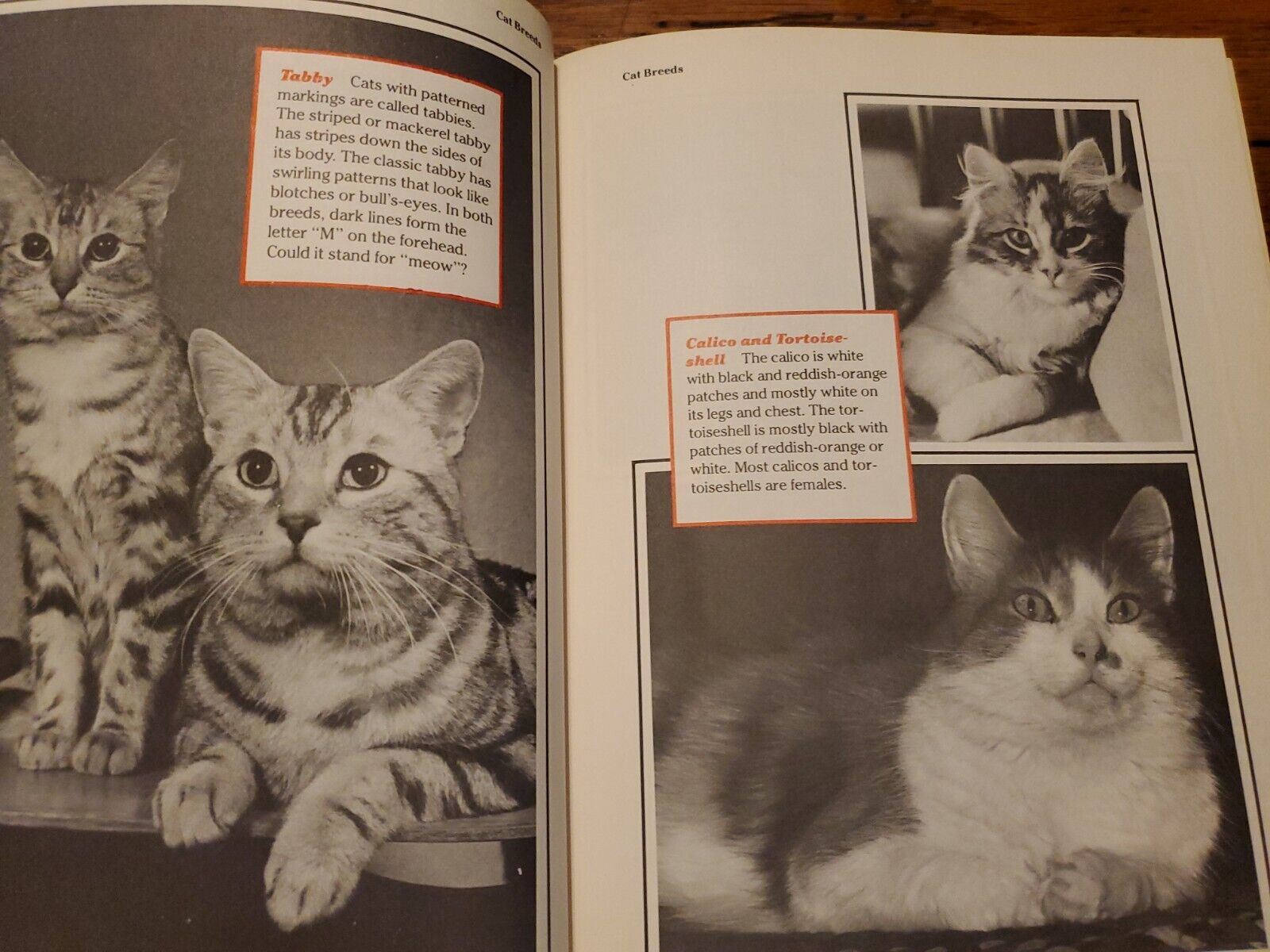The image reveals an overhead shot of an open book titled "Cat Breeds," featuring black-and-white photographs and detailed descriptions of various types of cats. On the left page, there's a full-page photograph of two Tabby cats, one sitting up and the other lying down and looking away. Surrounding the picture, red markings accentuate the text box, with a red title that reads "Tabby." The accompanying text explains that tabby cats are characterized by pattern markings, and it describes different types: the striped or mackerel tabby, with its distinct side stripes, and the classic tabby, with its swirling patterns resembling blotches or bullseyes. Both types feature dark lines on their foreheads forming an "M," which whimsically might stand for "meow."

The facing right page presents two more black-and-white photos of cats, designated as Calico and Tortoiseshell. The descriptive text elaborates that calico cats are predominantly white with black and reddish-orange patches, often exhibiting more white on their legs and tail. Tortoiseshell cats, on the other hand, are primarily black with patches of reddish-orange or white. Both calicos and tortoiseshells are predominantly female. The crisp, black-and-white images combined with detailed captions create an informative and visually engaging segment of the book.